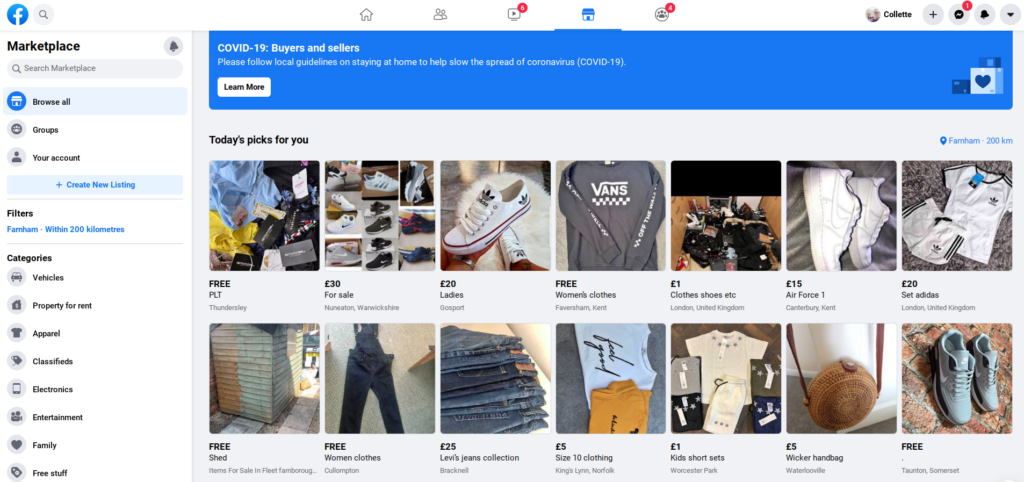This is a detailed screenshot from a Facebook browser window, showcasing the Marketplace section. The left sidebar features multiple elements, starting with a header titled "Marketplace" that includes a search bar below it. Adjacent to the search bar, aligned to the top right within the sidebar's boundaries, is a bell icon. The sidebar is organized into several sections: 

1. **Navigation:**
   - Highlighted in blue, "Browse All" is the first row indicating the currently selected option.
   - Followed by "Groups" and "Your Account."
   - Below these, there is an option labeled "+ Create New Listing."

2. **Filters:**
   - This section specifies "Within 200 kilometers," indicating the geographic filter applied to the search results.

3. **Categories:**
   - This is the third section of the sidebar, but specific categories are not detailed in the provided description.

The central and larger part of the webpage features a prominent blue banner at the top that reads, "COVID-19: Buyers and sellers, please follow local guidelines on staying at home to help slow the spread of coronavirus COVID-19." There is also a "Learn More" button presented in white.

On the right pane, the display title is "Today's Pick For You," showcasing two rows of items, primarily clothing articles and shoes. Details of the items include:
- The first item in the top row is labeled "Free" and titled "Thunderslay."
- The second item in the top row is shoes listed for "£30."
- In the second row, the first item is a "Free" shed.
- At the top right corner of this section, there is a reference to "Farm Hand at 200 kilometers," which likely indicates a geographical filter applied to the displayed items, corresponding to a location within a 200-kilometer radius.